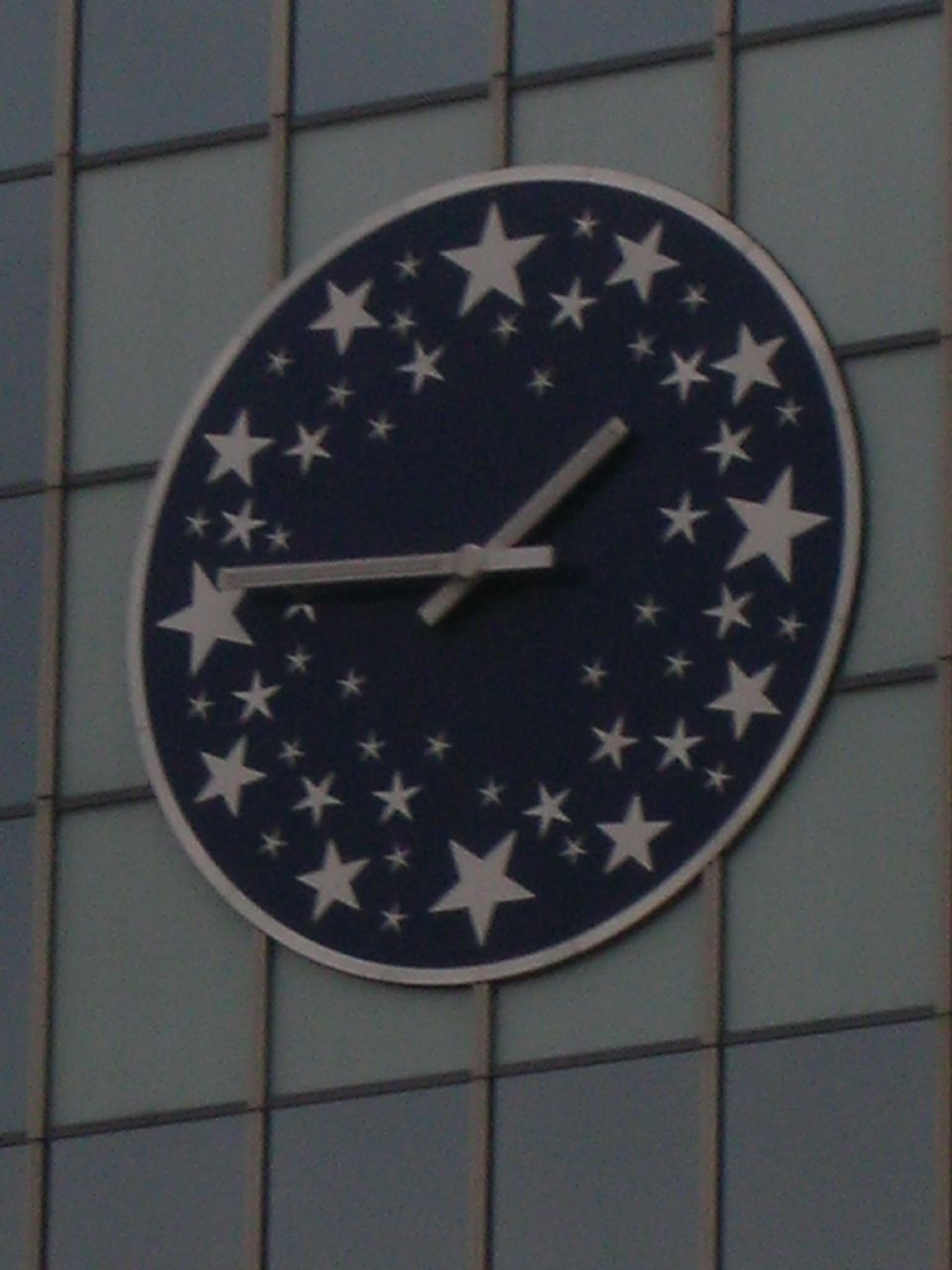The image depicts a large, analog clock with a circular face mounted on a building adorned with glass windows. The windows are square-shaped and vary between light blue to light teal in color, giving the façade a checkered appearance with alternating light and deep grayish-blue squares. In total, 12 light blue squares are clearly visible, bordered by the darker squares.

The clock itself features a dark blue, almost navy background. Its face is decorated entirely with silver stars instead of numerals. Prominent larger stars are positioned where the numerals 12, 3, 6, and 9 would typically reside, while smaller stars fill in the positions for the remaining hours, creating a celestial theme. The time displayed on the clock is approximately 1:47. The clock hands, made of metal, stand out with a sleek, stainless steel finish. The unique combination of the clock's design and the building's striking windows makes for a captivating and detailed visual.